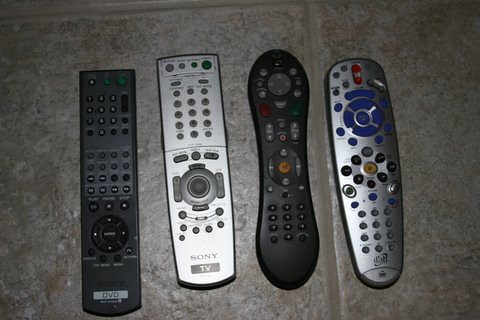The photograph depicts four remote controls of varying shapes and colors laid out horizontally on a grey tile floor with lighter grey grout lines visible between them. On the far left is a black remote control labeled "DVD" at the bottom, featuring black buttons. To its right is a silver remote control with the inscription "Sony" followed by "TV" beneath it, and it is equipped with gray buttons. The third remote control from the left is black, with white buttons at the top and black buttons at the bottom, but it lacks any visible labels. The fourth and final remote control on the far right is silver, notable for its colorful buttons that include red, blue, yellow, black, and grey. It has a blue circular area at the top, additional black buttons, a distinct yellow button, and the brand "DISH" outlined in black at the bottom. The remote controls are of different shapes, with some being more rounded and others wider at the top and narrower at the bottom, and they all appear to be older models.